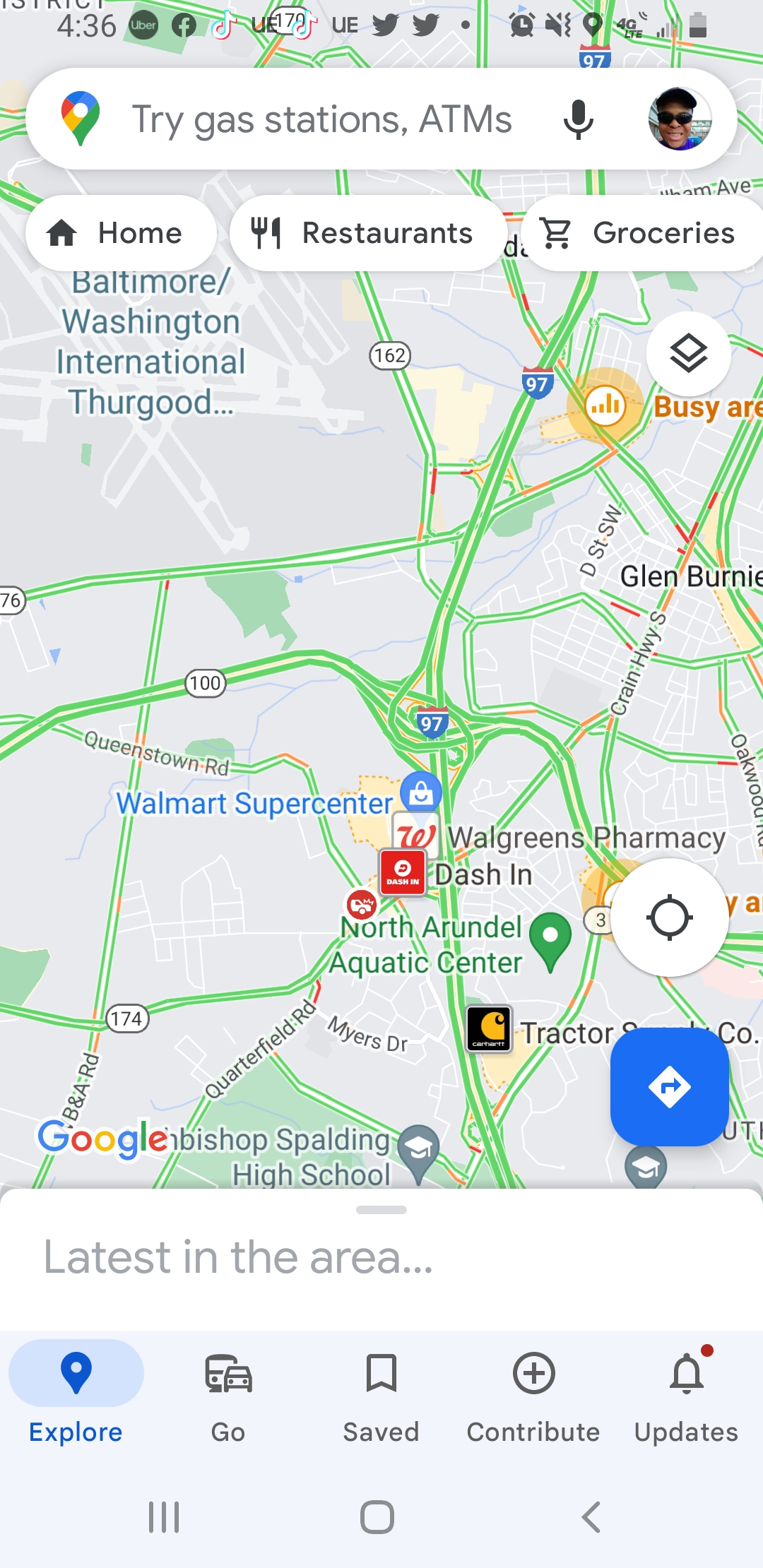Screenshot of a Google Maps view featuring multiple notification icons across the top bar, indicating that Facebook, TikTok, Twitter, an alarm clock, sound settings, and location services are active. The map displays a detailed section of Baltimore-Washington International Thurgood Marshall Airport on the left. Central to the image is a significant intersection involving Interstate 97, intersecting with Route 100. Notable landmarks include Walgreens Pharmacy, Dashion, and the North Arundel Aquatic Center situated in the middle section. In the bottom right corner, a Carhartt logo is visible, along with a Tractor Supply Company store marker. The bottom left corner prominently features a Google logo. At the very bottom of the interface, the 'Explore' tab is highlighted, alongside other options such as 'Go,' 'Save,' and 'Contribute.'